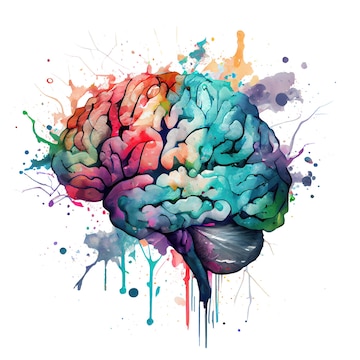The image features a detailed black ink drawing of a human brain, centered against a white background. This monochrome depiction is vividly contrasted by a vibrant array of colored ink splotches that resemble paint splatters. Colors include green, gray, red, purple, turquoise blue, orange, and various mixed hues forming a grayish blue-black tone. The splotches appear randomly distributed, with some ink visibly dripping down across the cerebrum towards the bottom of the picture. The blend of colors creates a rainbow-like effect, contributing to an overall impression of a digital art piece reminiscent of watercolor techniques. This artistic rendering also exhibits some cracks in the background, enhancing its textured appearance.